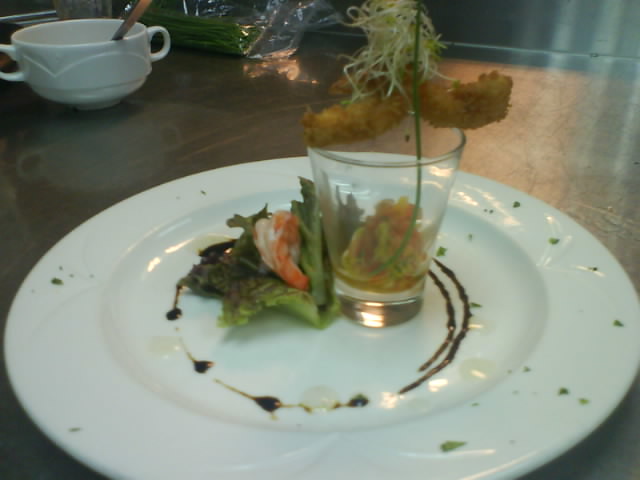The image depicts a detailed and artfully presented dish, likely from a high-end restaurant, set against a kitchen backdrop indicated by a pot and a plastic bag seen in the background. The focal point is a meticulously arranged white plate centered in the image, adorned with a small, vibrant salad and a shrimp. The plate is artistically decorated with green drizzles and dark circular sauce patterns. Adjacent to the plate is a small glass cup containing shrimp and possibly tomato elements, crowned with fried shrimp and a sprinkle of parsley. The setting is brightly lit, highlighting the dish's intricate presentation and vibrant colors against the backdrop of a preparation area.